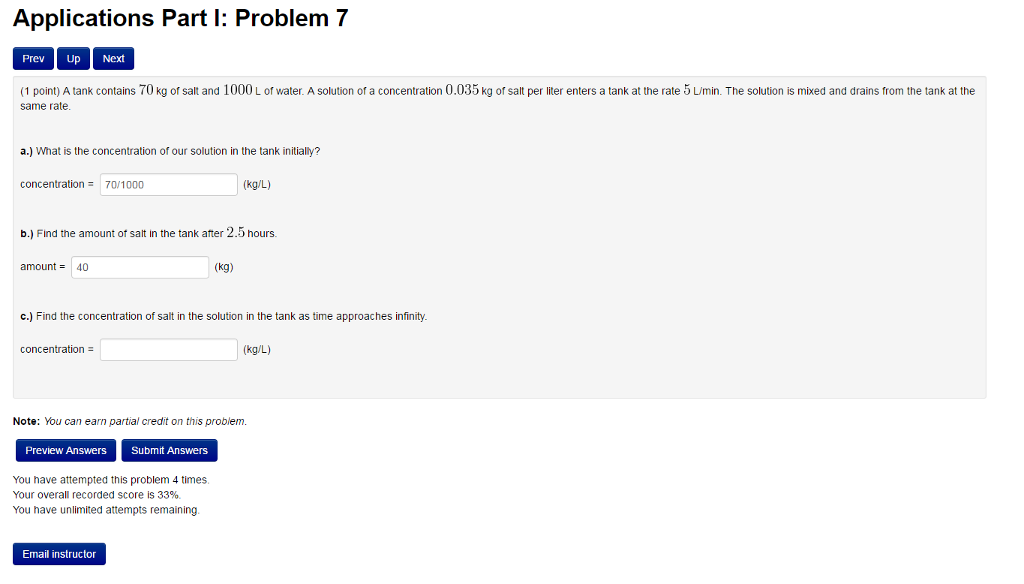**Image Description: Complex Problem Explanation Interface**

The image depicts a page with a predominantly white or gray background. At the top of the page, the title "Applications Part 1: Problem 7" is displayed. On the left side, there are navigational buttons labeled "Previous," "Up," and "Next" in blue with white text.

Below these buttons, the page content is divided into sections. The first section features a problem description on a gray background with black text. It states:

"1. (a) A tank contains 70 kilograms of salt and 100 liters of water. A solution with a concentration of 0.035 kilograms of salt per liter enters the tank at a rate of 5 liters per minute. The solution is mixed and drains from the tank at the same rate. What is the initial concentration of the solution in the tank? The concentration is given by 70/1000 kg per liter. (b) Find the amount of salt in the tank after 2.5 hours. The amount is 40 kilograms. (c) Find the concentration of salt in the solution in the tank as time approaches infinity. The concentration is ______ (data field with no answer)."

Additionally, the problem notes that partial credit can be earned for correct parts of the solution.

Towards the bottom, there are two buttons labeled "Preview Answers" and "Submit Answers," both in blue with white text. Below these buttons, the page informs the user: "You have attempted this problem 4 times. Your overall record score is 33%. You have unlimited attempts remaining. Email instructor."

Each of the data fields provided for answers has corresponding answers filled in, except for the last one which remains empty.